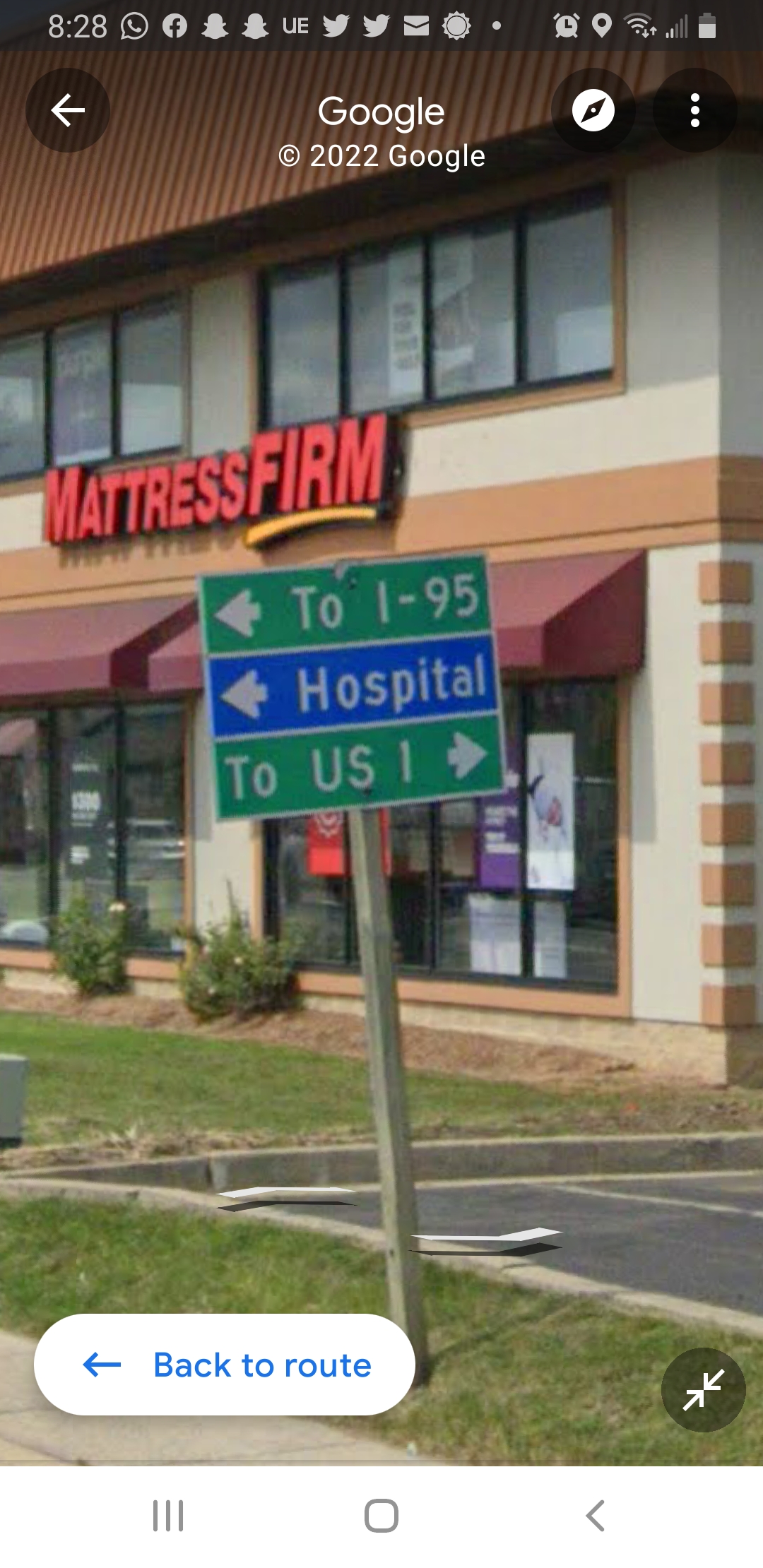The image appears to be a screenshot from a mobile phone, likely captured from within a navigation application. The primary focus is a street view showing a Mattress Firm store in the background. In the foreground stands a street sign on a pole, displaying multiple directional arrows and routes. The sign points left towards I-95 and the hospital, and right towards US-1. 

At the top of the screenshot, the time is displayed as 8:28, along with the Google logo and a footer notation indicating "2022 Google." The bottom of the screen features a white rectangular button with a blue left-pointing arrow and the text "Back to route." 

Additionally, the screenshot shows various status icons at the top, including emblems for Facebook, phone calls, Snapchat, Twitter, a clock, Wi-Fi connectivity, and battery power status.